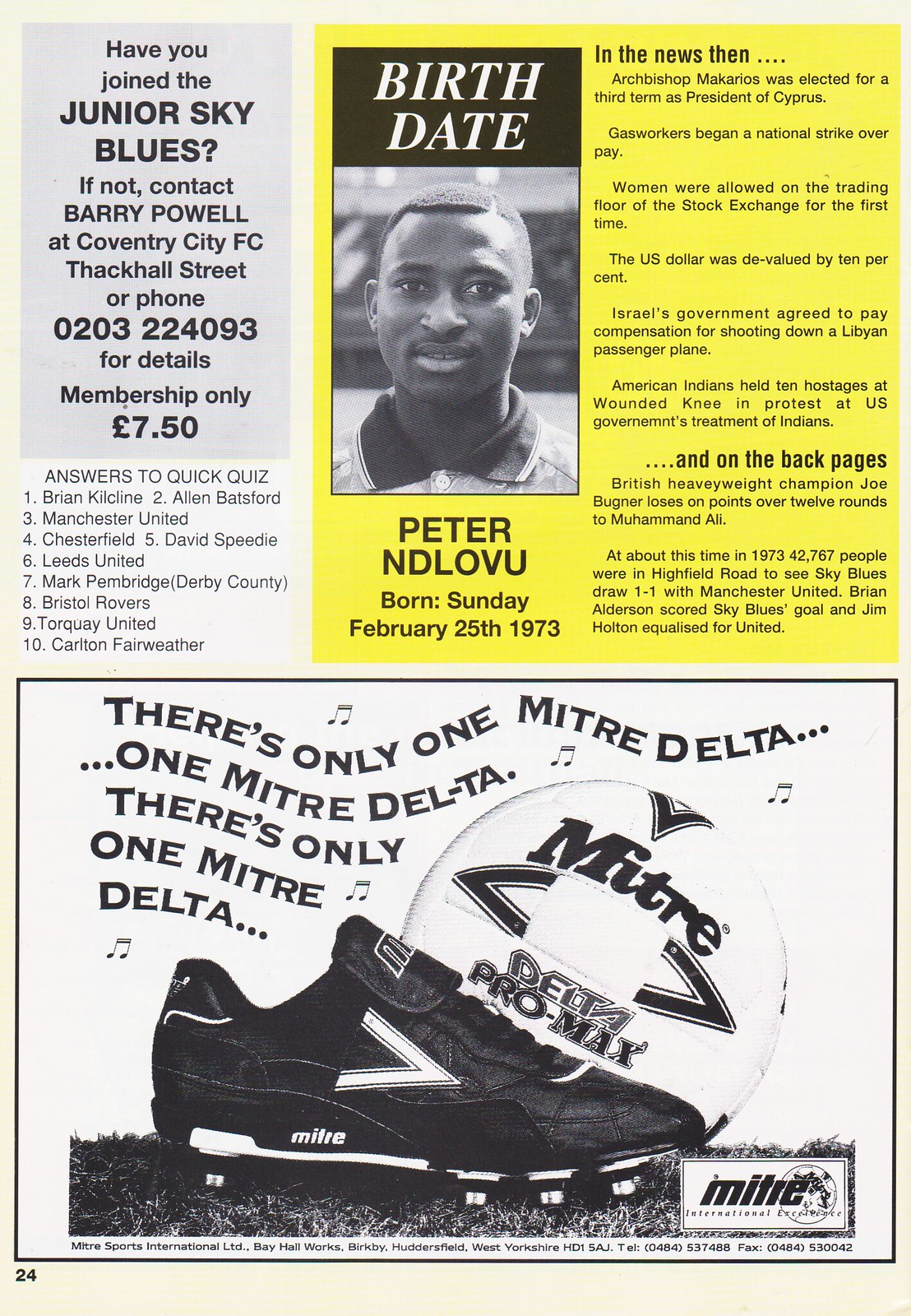The image showcases a magazine flyer featuring a prominent soccer player and an advertisement dedicated to soccer enthusiasts. The top left corner contains a small rectangle with a black text invitation encouraging readers to join the "Junior Sky Blues" by contacting Barry Powell at Coventry City FC, Thackall Street, or by calling 0203-224093. Membership is listed at only £7.50. Adjacent to this, on a yellow background square, there’s a portrait of a man in a collared button-up shirt. 

At the bottom of the image, a soccer cleat is pictured sideways next to a soccer ball, accompanied by the repetitive slogan, "There's only one Major Delta." These items in the advertisement aim to attract attention with a rhythmic phrase. Towards the top, various black and white text blocks deliver additional details and advertisements. One of the key highlights is a black and white photo of Peter Ndlovu, with the text beneath detailing his birthdate as Saturday, February 25, 1973. The overall composition of the flyer combines text-heavy information with visual elements, making it an engaging promotional piece for soccer fans and potential Junior Sky Blues members.